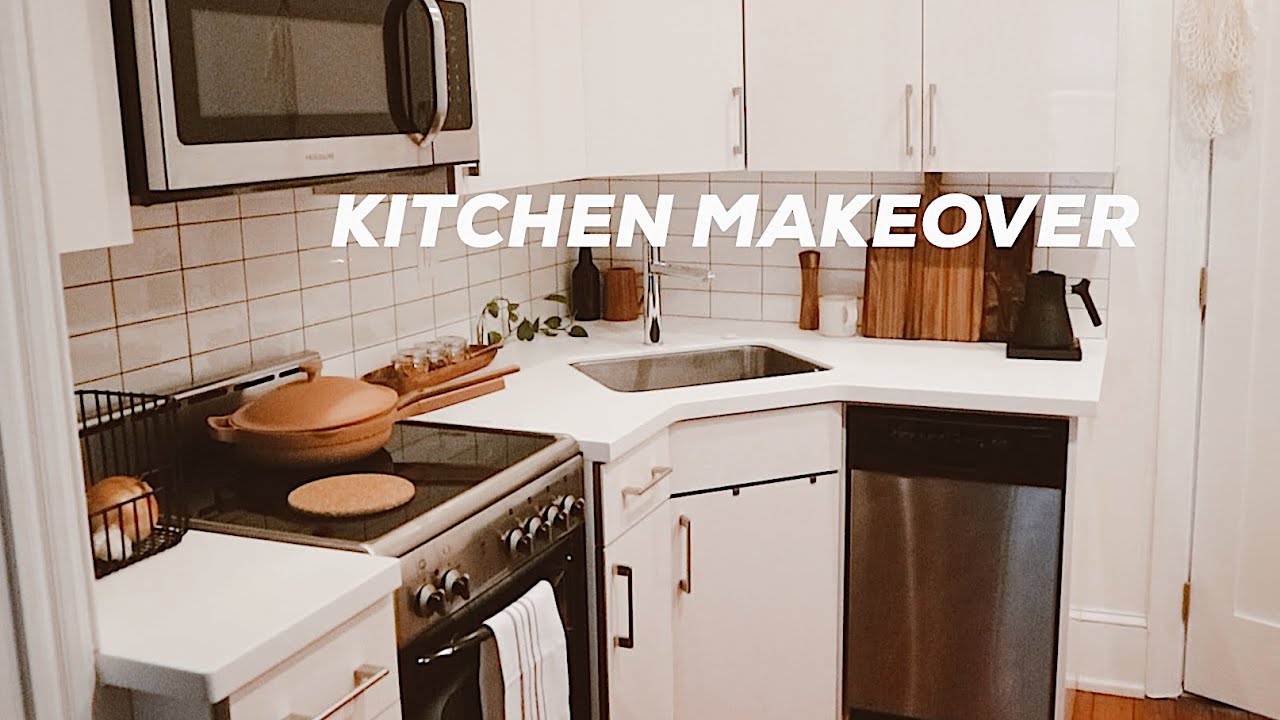The image showcases a professionally done kitchen makeover in a compact corner galley layout. Bold, bright white text in the center of the image reads "Kitchen Makeover." The space is efficiently designed with white cabinets wrapping around the available area, and a white tiled backsplash enhancing the bright aesthetic. A small, aluminum-and-black two-burner stovetop sits just to the left of a tiny sink, with a microwave and hood positioned above. Several cabinets flank the microwave and continue to the right above the backsplash. Below, the limited counter space accommodates a very small dishwasher to the bottom right.

Accents include a teapot, a few dishes, and wooden utensils for staging. A door to the right, partially open and painted white, leads out of view. The kitchen features wood laminate flooring, adding a touch of warmth. Despite its pretty appearance, the kitchen feels cramped and impractical for extensive cooking, especially with the limited space and presence of an onion basket, a plain cheese board, a cork placemat, a striped white drying towel hanging from the oven, various spices, and a small dish placed between the sink and the stove. The overall scene suggests a before image, capturing the challenges of working in such a confined space.